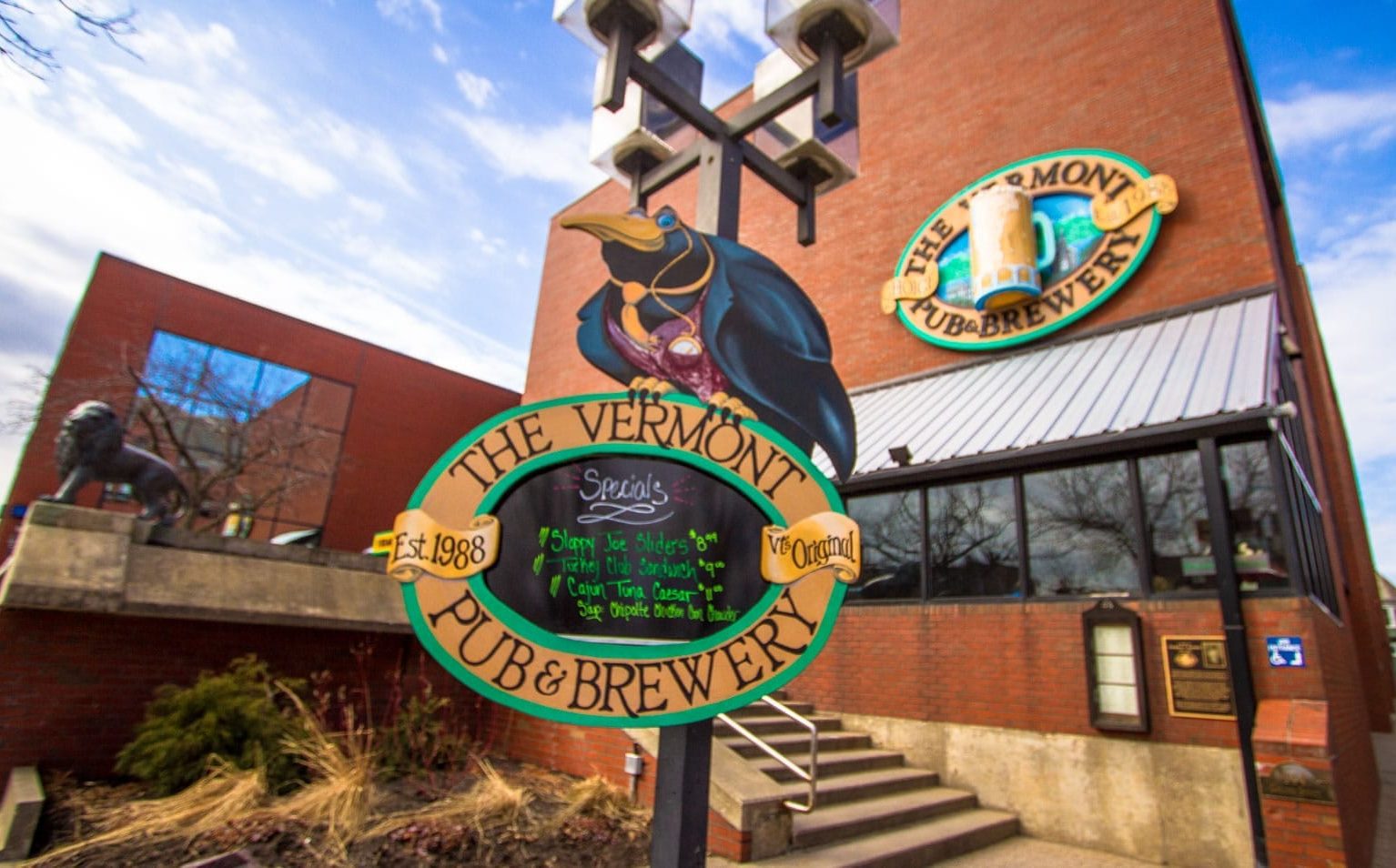This image beautifully captures the entrance of the Vermont Pub and Brewery, established in 1988, on a bright day with a clear blue sky dotted with white clouds. The pub, housed in a red brick building with a gray staircase leading up to the entrance, displays a large sign in front. This sign advertises the daily specials: Sloppy Joe Shades for $8.99, Turkey Club Sandwich for $9, and Cajun Tuna Caesar for $8, written in light green against a white background with whimsical squiggles underneath. The pub's sign above this features a prominent crow dressed in a black suit, yellow tie, red vest, yellow beak, black claws, and blue eyes, perched atop, adding a quirky charm to the scene. Additional details include a 3D beer mug displayed in the pub's logo, visible conservatory-like glass windows, and a silver railing along the concrete steps. Enhancing the exterior view, there's some lush, green shrubbery on the left side at the bottom of the steps, and a majestic iron lion statue at the top. The image emphasizes the Vermont Pub and Brewery's inviting and distinctive facade, a testament to its established heritage and unique character.